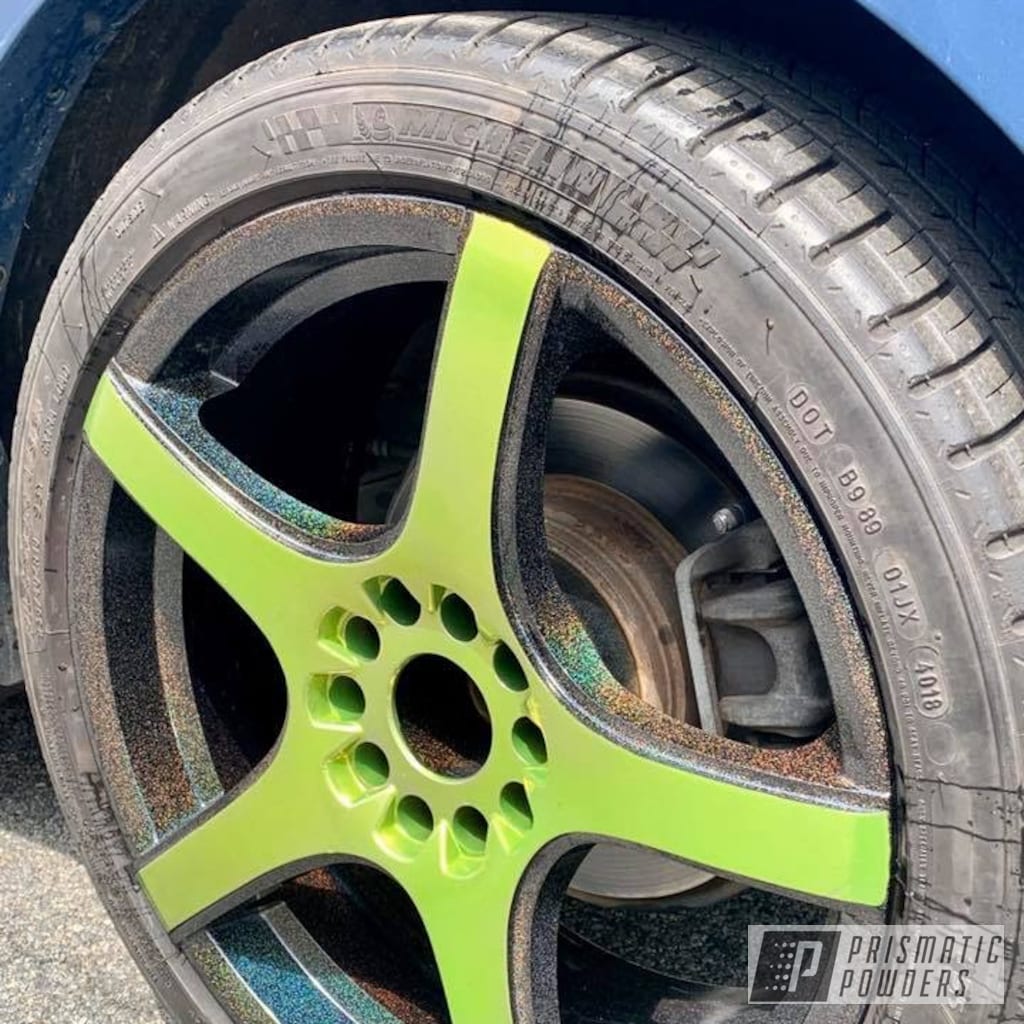The image captures a close-up view of a worn Michelin tire on a blue car, showcasing just the tire and parts of the vehicle's brake system. The zoomed-in perspective crops out the bottom of the tire, and only small sections of the car are visible in the top corners, confirming its blue body. Central to the composition is a rusted five-pointed star-spoked rim, strikingly painted with a vibrant lime green color using prismatic powders, creating a bold contrast with the rust and adding splashes of yellows and reds from dye bleeding. The intricate detailing includes a printed stylized 'P' in the lower right-hand corner, and inscribed text ".B98901JX4018" can be seen on the tire's wall. The image serves to highlight the wheel's artistic and functional elements, from the star-shaped spokes to the visible brake pads and components behind them.